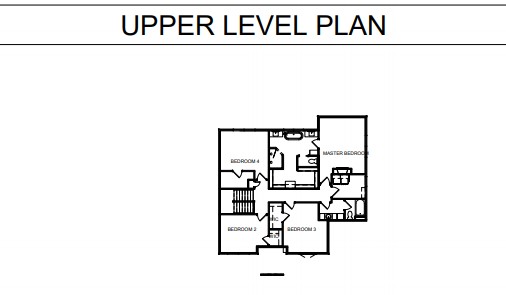This diagram depicts the upper-level floor plan of a spacious home, as indicated by the "Upper-Level Plan" label prominently displayed at the top in black lettering. The architectural layout, meticulously drawn with black ink and ruler, outlines a large upper floor divided into multiple rooms. Notably, the plan includes three standard bedrooms labeled as Bedroom 1, Bedroom 2, and Bedroom 3, alongside a more substantial Master Bedroom, suggesting a sizeable residential space. 

Although the specific functions of some areas are not labeled, the layout clearly delineates all rooms and passageways. The diagram also identifies the locations of restrooms, a stairway leading downstairs, and hallways that connect the various living spaces. The master bedroom features its own dedicated bathroom, while another bathroom services the three adjacent bedrooms. This clear, precise architectural drawing offers a comprehensive view of the upper-level layout, showcasing the thoughtful distribution of living spaces typical of a large home.